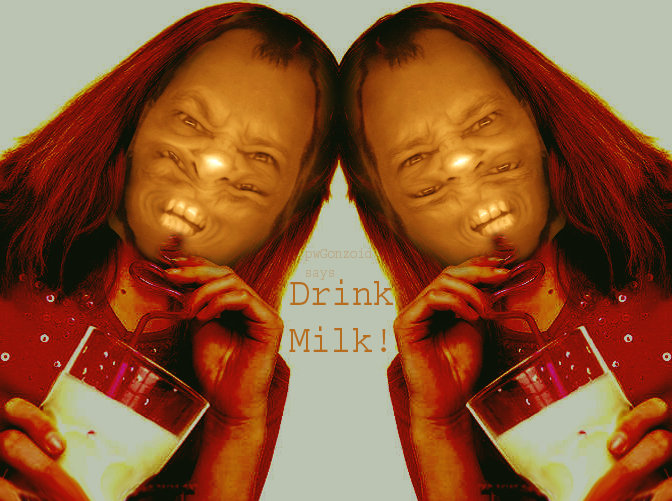This advertisement features the distorted, mirrored image of a person, digitally altered to appear monstrous, with a yellowish-brown face and exaggerated features. The figure's eyes are doubled, creating the illusion of four eyes, their nose is rounded and centralized, and their bared teeth are accentuated with stretched lines at the mouth's sides. The person, who has red hair, wears a red shirt with a slight V-neck and white circles, and holds a glass of milk in one hand and a pink or purple crazy straw in the other, though not actually drinking from it. At the center of the poster, in large dark text, the phrase "DRINK MILK!" is prominent, with a faded, small orange text above it that reads "PWGONZOID says," emphasizing the playful and surreal nature of the image.